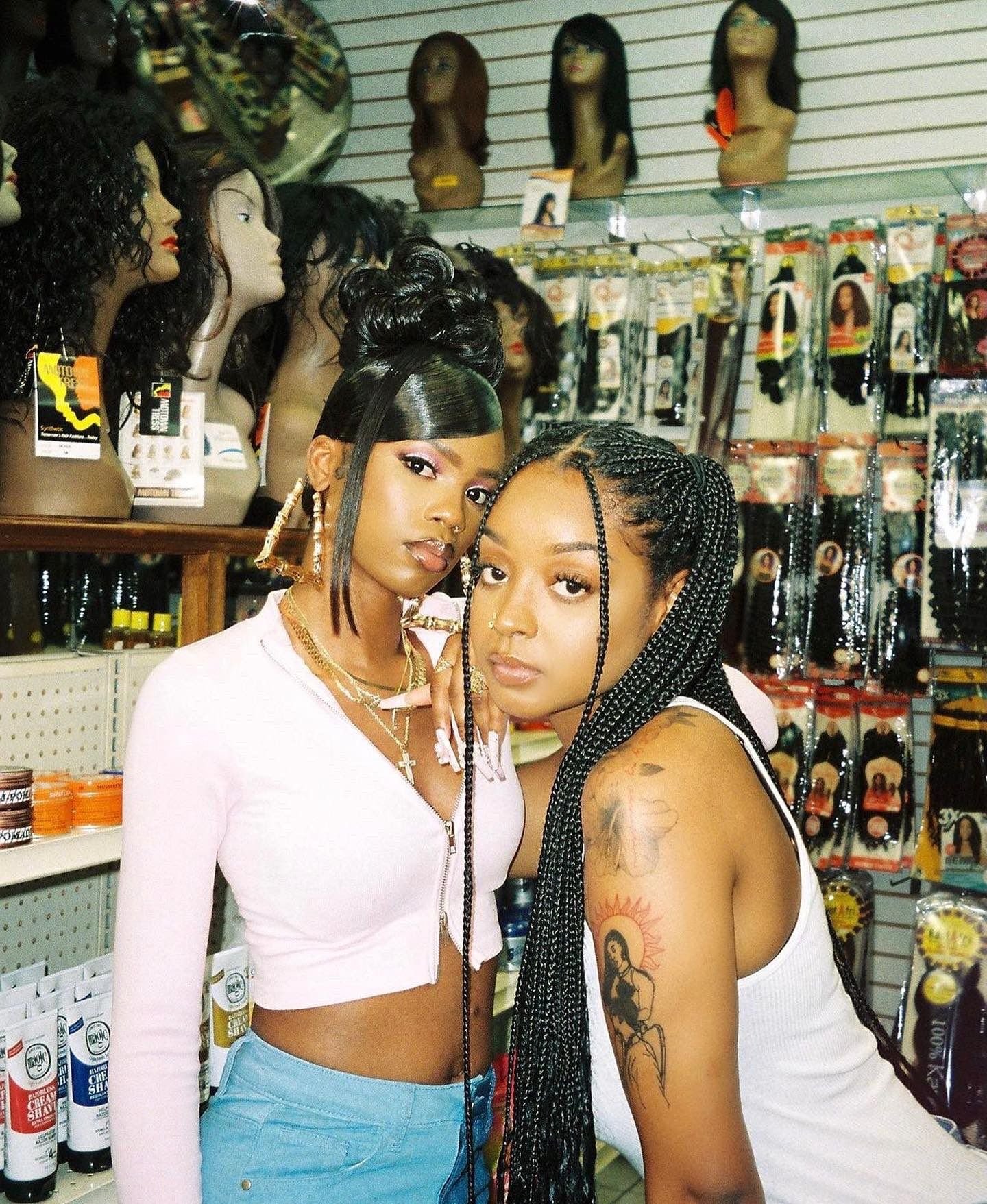In a vibrant beauty shop filled with mannequins showcasing an array of wigs and hair products, two petite, stylish African-American women pose for the camera. Both women exude confidence and elegance, sporting distinct yet equally captivating hairstyles. 

The woman on the left wears a fitted white crop top with full sleeves and a zipper, revealing her toned midriff and blue jeans. Around her neck, she flaunts a golden cross pendant complemented by humongous triangular gold earrings, and a nose ring. Her silky smooth hair is intricately styled in a flower-shaped bun, enhancing her attractive makeup and expressive eyes.

Beside her, the second woman stands out with her long, meticulously braided hair cascading out of the frame. She dons a ribbed, white racerback tank top that accentuates her fit physique. Her arms are adorned with detailed tattoos, including a striking image of a woman with a sun and a flower. Both women, leaning slightly into the shot, exude a sense of poised fashion forwardness, perfectly framed against the background filled with rows of hair care products, creams, gels, and mannequins.